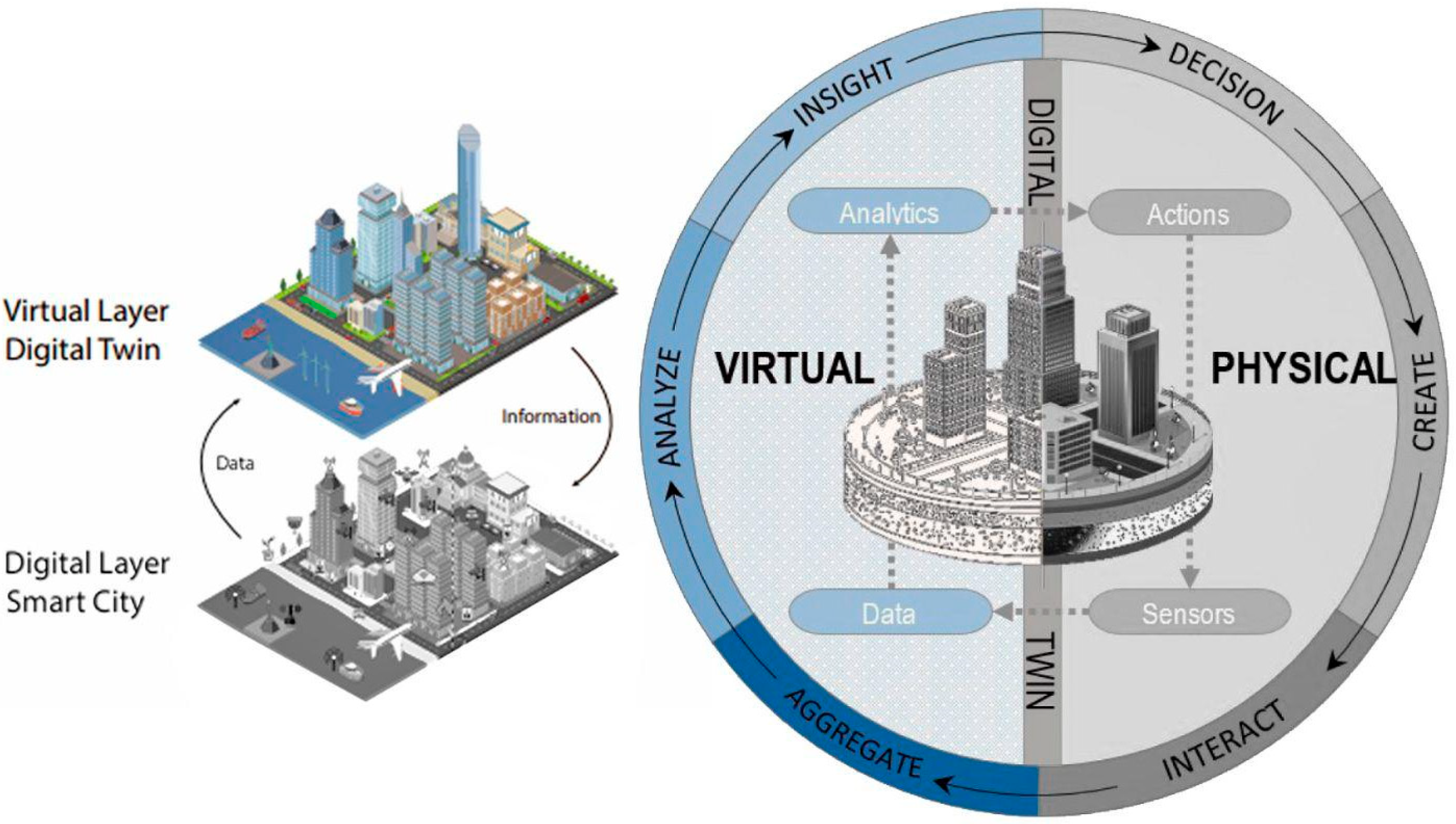The image is an intricate infograph showcasing a digital twin of a smart city. On the left, it features two versions of a cityscape: a colorful rendered drawing labeled "Virtual Layer Digital Twin" and a black and white version labeled "Digital Layer Smart City." Connecting these versions are two arrows, with the arrow pointing to the colored city marked "data" and the one pointing to the monochrome city marked "information." The colors used in the design include red, white, blue, black, gray, pink, green, brown, and orange.

Adjacent to this, a circular chart illustrates a dynamic cycle. This circle, divided into shades of blue and gray segments labeled with steps such as "Decision," "Create," "Interact," "Aggregate," "Analyze," and "Insight," forms a continuous loop indicative of the decision-making process. At the center of this chart, a vertical line divides it into "Virtual" on the left with a dotted cityscape, and "Physical" on the right with a more solid rendition of the city. Along this line, the term "Digital Twin" appears, highlighting the integration of virtual and physical elements. Additionally, within the cycle, ovals labeled "Analytics," "Actions," "Sensors," and "Data" are interconnected, demonstrating a flow of information between these components.